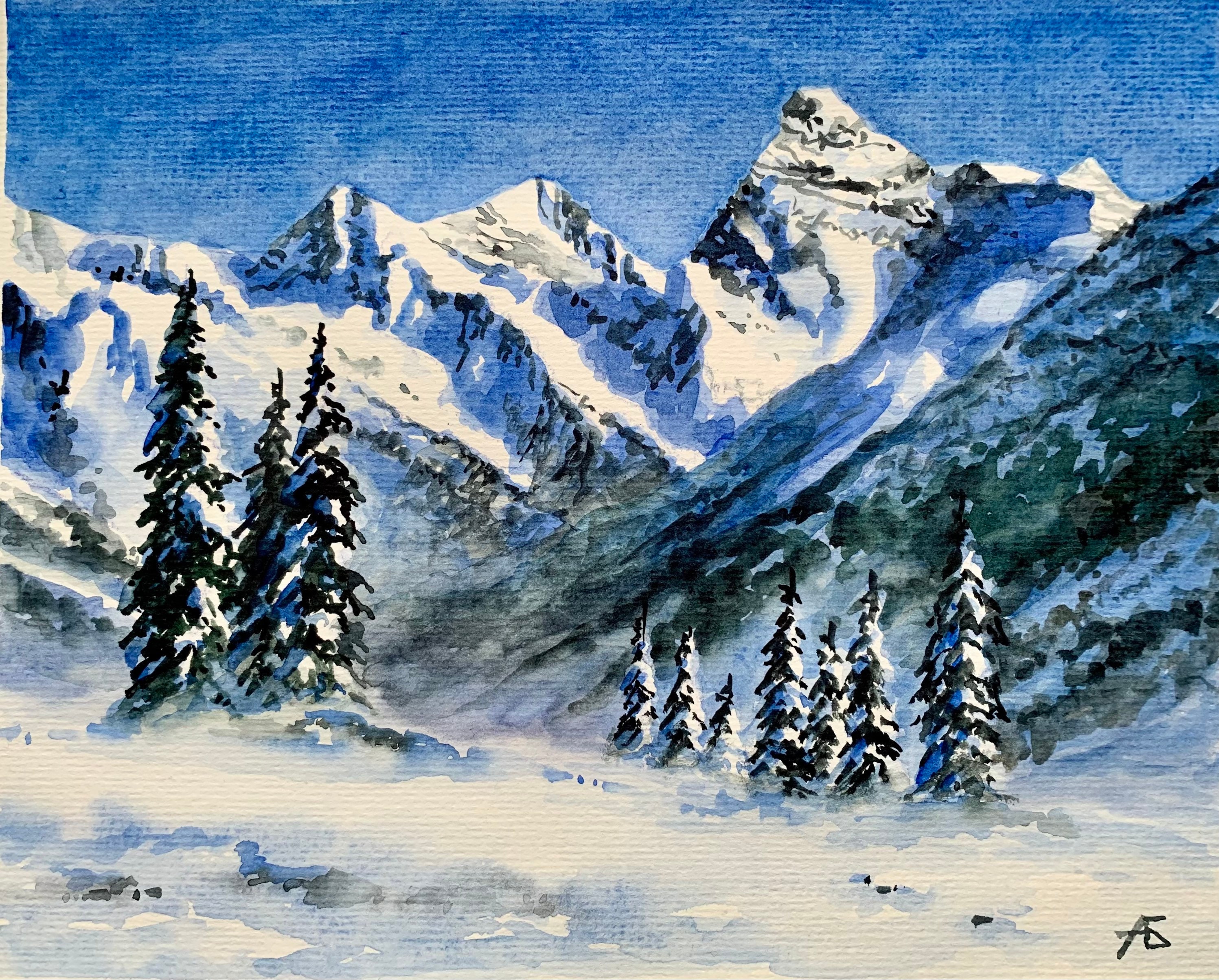This captivating painting showcases a serene winter landscape with remarkable detail. Dominating the scene is a dramatic dark blue sky, providing a striking contrast to the snow-clad mountains. The mountains are rendered with intricate precision, featuring an array of towering peaks and deep valleys, all blanketed in fresh snow. Tall, pointed evergreen trees punctuate the landscape, their boughs heavy with snow yet still revealing patches of vivid green needles. The ground beneath is similarly cloaked in snow, but small grayish areas signify spots where the snow has receded, exposing rocks and earth. These dark rocks peek through the snow, adding texture and depth to the tranquil scene. The thoughtful interplay of colors and elements creates a vivid, almost palpable sense of a winter wonderland.